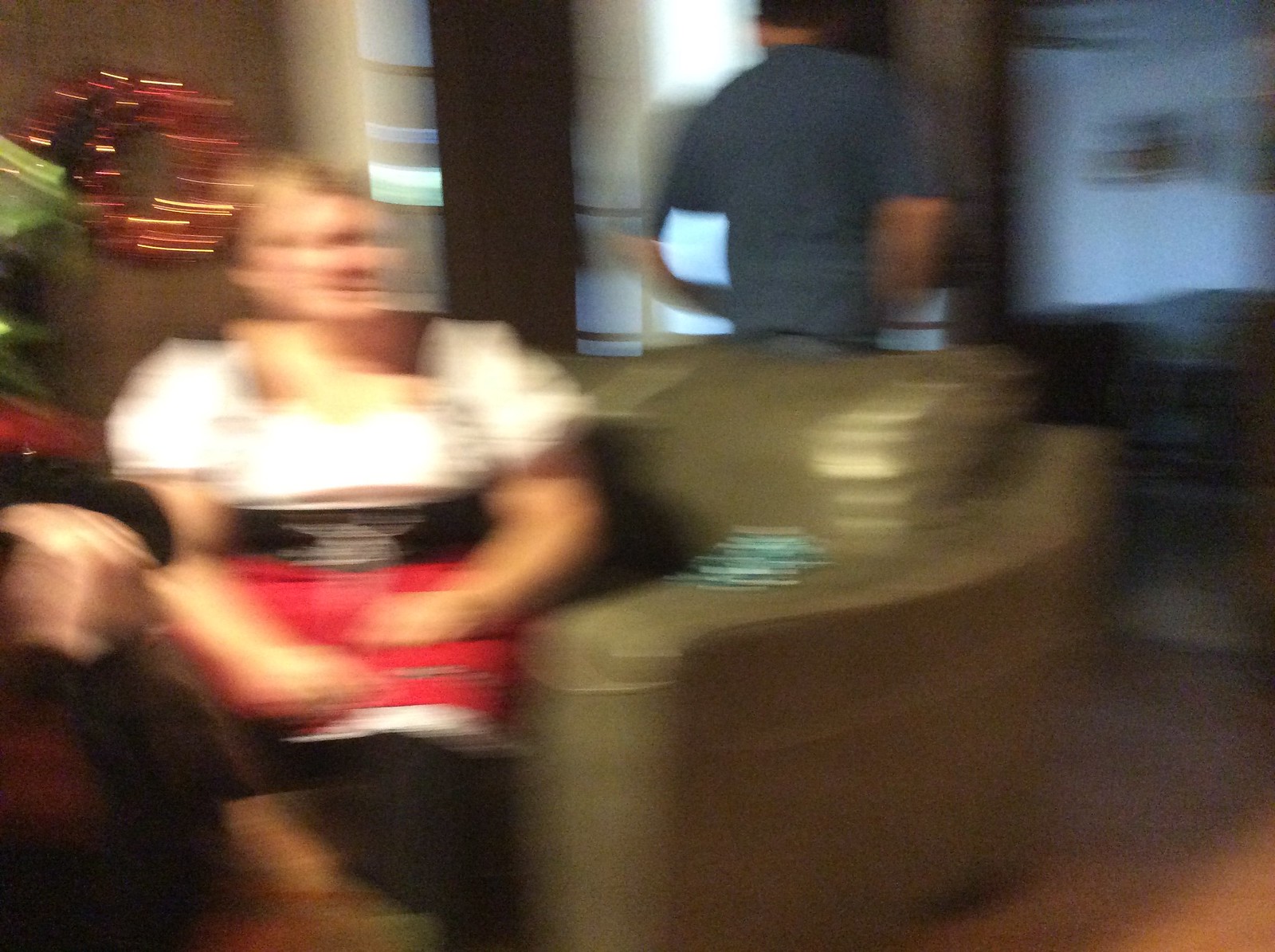In a blurry photograph depicting a cozy living room scene during Christmas time, one can make out festive decorations, including a red wreath adorned with lights on the left-hand back wall and a glimpse of a Christmas tree. In the foreground, a woman with blonde hair pulled back, fair skin, and wearing a dirndl skirt sits on a light brown chair or loveseat. Her attire includes a blouse with voluminous white puff sleeves and a square neckline, paired with a red skirt. Her hands rest in her lap, though the lower part of her outfit remains obscured, potentially hinting at black pants or a black skirt. Behind the couch, a man with dark hair, dressed in a short-sleeved blue-gray t-shirt, faces away from the camera with his hands positioned in front of him. The background shows another room to the right, but the details are indistinct.